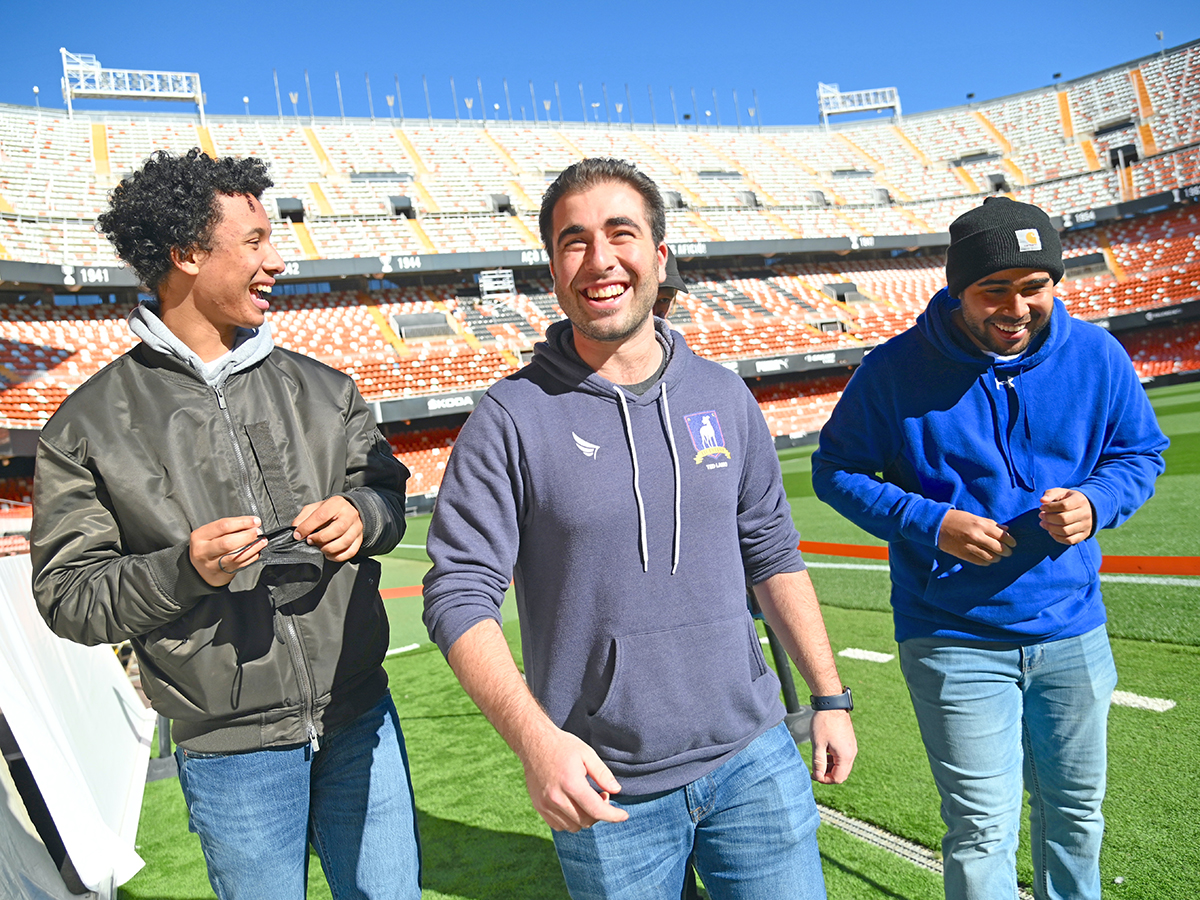This is a detailed photograph capturing a lighthearted moment with three men standing on the green astroturf of an empty American football stadium. In the center stands a white man with dark brown, slicked-back hair, and a relaxed smile. He is dressed in a gray hoodie with a front pouch and blue jeans, sporting a black wristwatch on his left hand. To his left, an African American man with curly hair is facing him, partially in profile. He wears a black or brown bomber jacket zipped over a gray hoodie, accompanied by blue jeans. To the right, another man is laughing, slightly hunched over with cheer. He is outfitted in a blue fleece hoodie, light blue jeans, and a black beanie with a white logo. The background reveals multiple rows of empty seats and a clear, cloudless blue sky, enhancing the sense of camaraderie and openness in the scene. The image conveys a relaxed and joyful atmosphere among friends within the vast, empty stadium.